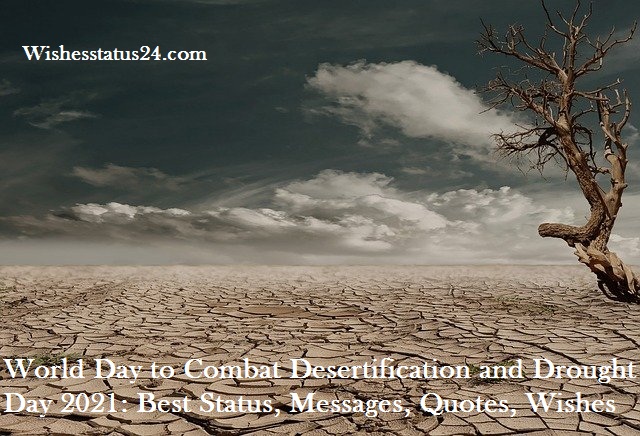The image depicts a stark, rectangular scene of extreme dryness. The upper 60% of the image features a dark blue sky dotted with white clouds, while the lower 40% reveals a parched, cracked desert landscape devoid of vegetation. Prominently located on the right side is a barren tree with a large trunk splitting into two sections midway up, completely devoid of leaves, encapsulating the lifelessness of the scene. Overlaid text at the top reads "wishesstatus24.com," and additional text towards the bottom states, "World Day to Combat Desertification and Drought, Day 2021. Best status, messages, quotes, wishes." The overall portrayal underscores the harsh impact of desertification and drought.